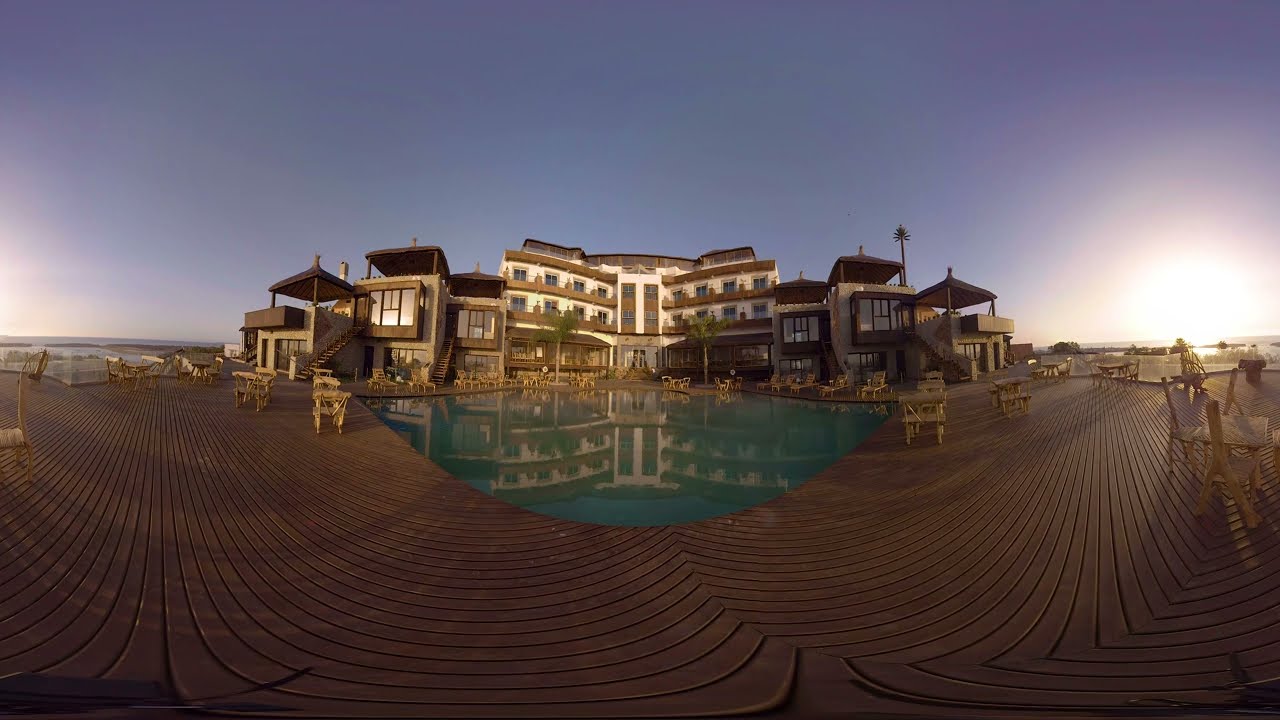The image showcases a large, four-story, beige house with brown trim that resembles a beach resort. Taken in panoramic mode, the picture is slightly warped, creating a mirrored effect on the left and right sides. The central structure features multiple balconies and double sliding doors at the entrance. On either side of this main building, there are staircases zigzagging up to decks adorned with large umbrellas. Surrounding the square, blue swimming pool in the foreground is a wooden deck with dark brown planks and an array of tables and chairs, approximately 15 in count, set up around the pool area. The serene setting is accentuated by the clear blue sky tinged with hints of purple, suggesting it is sunset. The sun is visible on the right side of the image, adding a warm glow to this beachfront retreat.